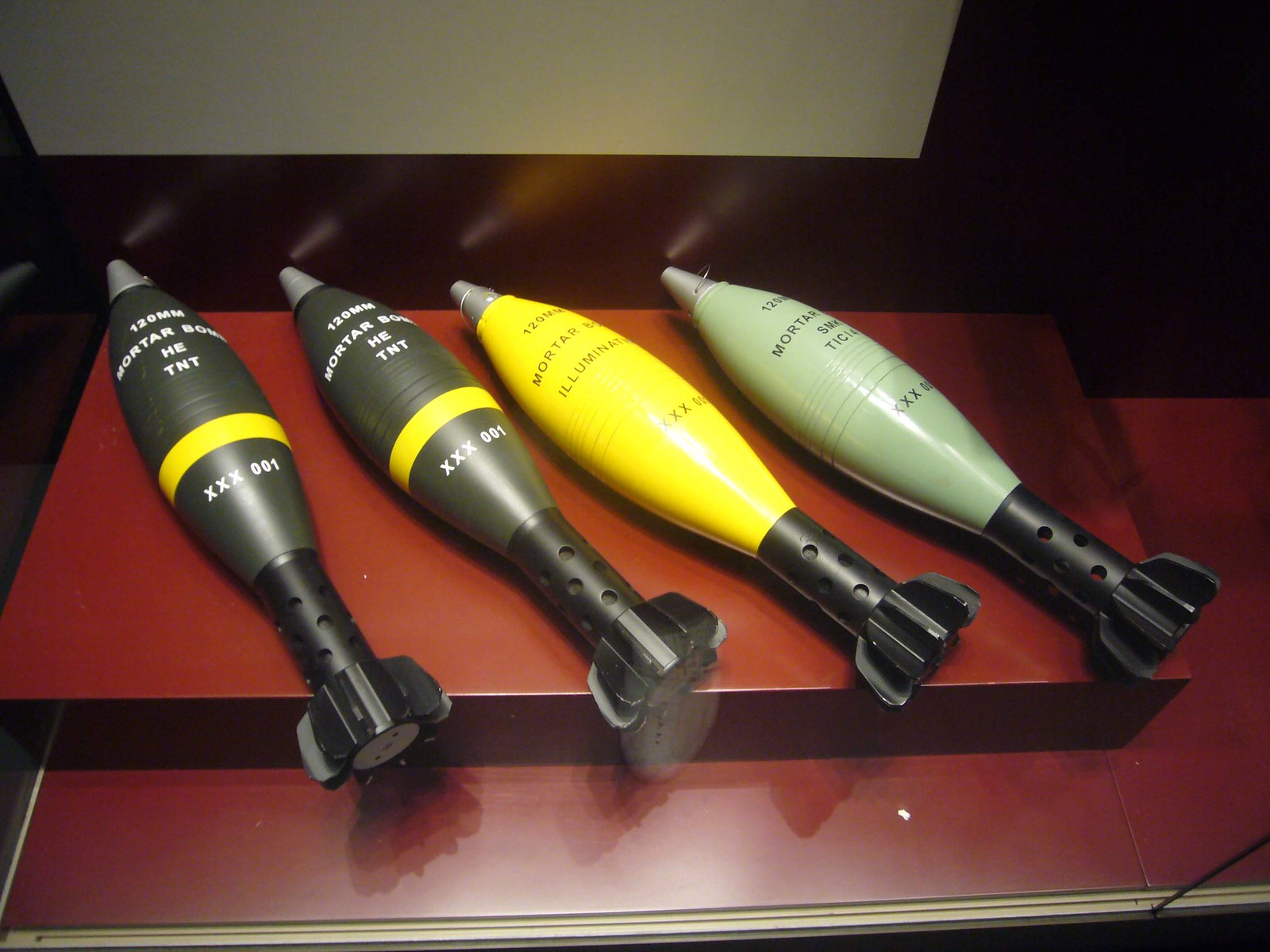The photograph captures an intricate display inside a war museum, showcasing four 120 millimeter mortar bombs, each with the marking H-E-T-N-T and labeled XXX-001. The mortar rounds are precisely arranged side by side behind a glass display case, positioned atop a striking burgundy-red podium. Each bomb is distinctly colored: the two on the left are in military green with yellow stripes, while the third is banana yellow and the fourth boasts a light turquoise hue. The mortar bombs, resembling rockets with a pointed tip, wide body, and narrow ending, provide an informative and visually compelling exhibit.